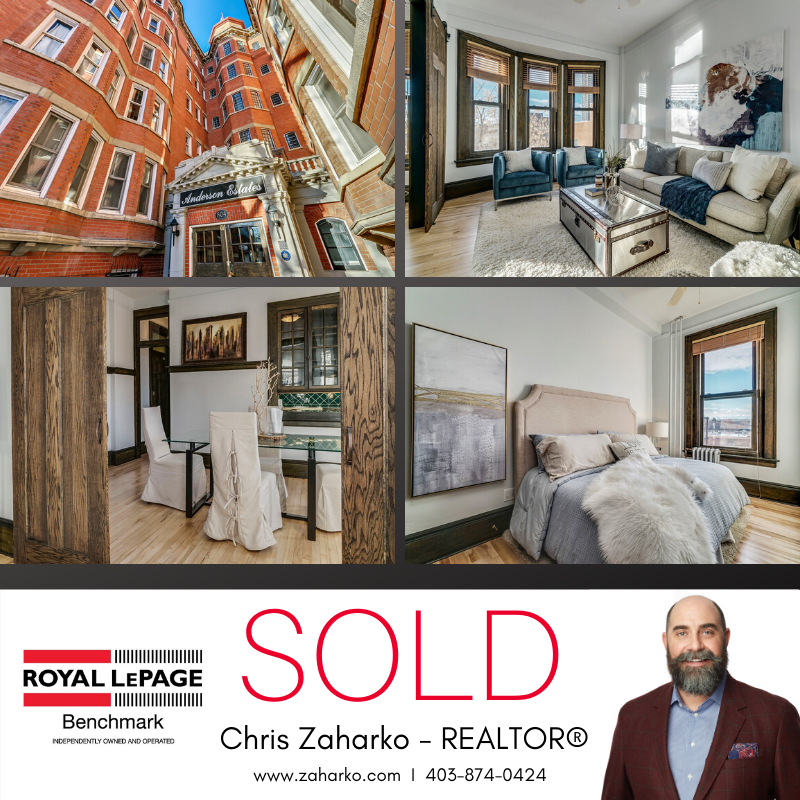This is an advertisement for the realtor Chris Zaharko, associated with Royal LePage Benchmark, an independently owned and operated firm. The ad features a large square divided into four smaller squares showcasing upscale property listings. 

- The top left image displays the exterior of an older, stately brick building.
- The top right image offers a glimpse into a stylish living room, likely from the aforementioned building.
- The bottom left image presents a sophisticated dining room, accentuated by wood flooring, chairs with fabric covers, and a glass dining table with black legs.
- The bottom right image shows a luxurious bedroom with a tan, upholstered bed. A large watercolor painting adorns the wall to the left of the bed. A round lamp stands in the corner, and a window with brown trim and a pulled-up wooden blind occupies the far wall.

At the bottom of the advertisement, the Royal LePage logo is prominently displayed, accompanied by the text, "Benchmark, independently owned and operated." Centered in the middle, large letters announce "SOLD" alongside Chris Zaharko's name and title as a Realtor. Below, the website www.zaharko.com and a contact phone number are provided.

On the right side of the ad, a professional photograph of Chris Zaharko is included. He is distinguished by his bald head, prominent facial hair, and mustache. He is dressed in a light blue button-up shirt, a maroon jacket, and a scarf tucked into the pocket.